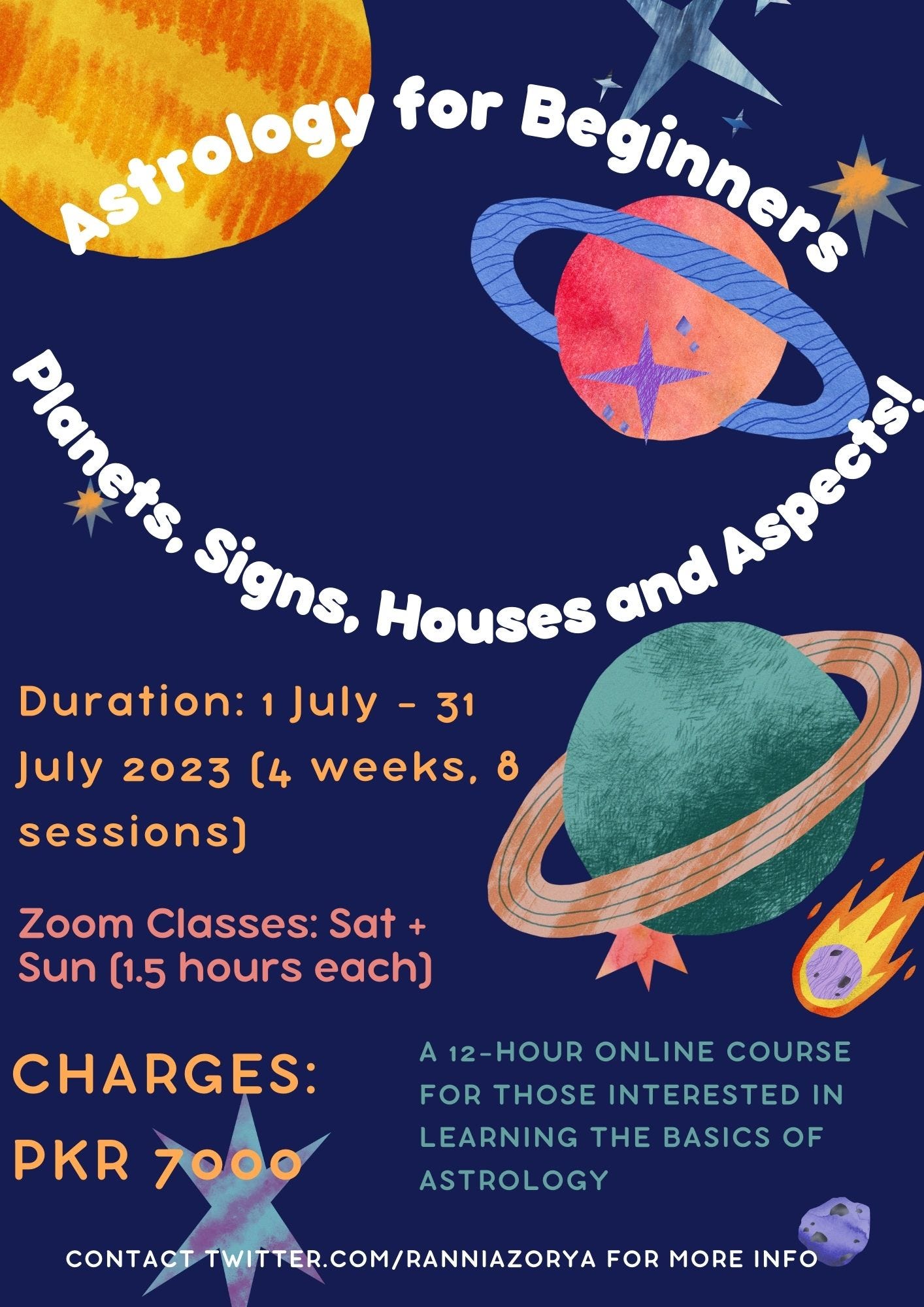The image is a detailed poster or flyer promoting "Astrology for Beginners." The entire background is a dark navy blue adorned with illustrations of planets, stars, and meteors. At the top, in large white text, it reads "Astrology for Beginners." Directly beneath this, in white text, it says "planets, signs, houses, and aspects." The course duration is listed on the left side in yellow text as "1 July to 31 July 2023," followed by "(4 weeks, 8 sessions)" in brackets. Below this, in red text, it mentions "Zoom classes Saturday + Sunday," with "(1.5 hours each)" in brackets next to it.

Below the course schedule, the charges are displayed in yellow: "Charges: PKR 7,000." Towards the right side of the poster, it states, "A 12-hour online course for those interested in learning the basics of astrology" in blue text. At the bottom, the contact information is provided in white text: "Contact twitter.com/RaniaZoria for more information." The background visuals include an orange and yellow orb representing the Sun, silverish-blue stars, a red planet with a purplish-gray ring, a green planet with bronze rings, and a purple meteor with flames.